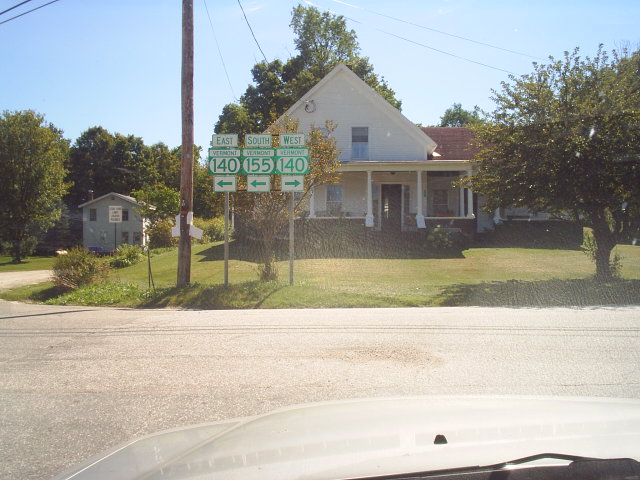This color photo, captured from the driver's seat of a tan sedan, shows a rural intersection in Vermont on a clear, sunny day. Prominently displayed ahead are three white street signs with green borders and text. The leftmost sign indicates "East Vermont 140" with an arrow pointing left, the center sign reads "South Vermont 155" also with a leftward arrow, and the rightmost sign points right to "West Vermont 140." Additionally, there is a modest, old ranch-style house with green foliage and a lush lawn, suggesting a summer setting. To the left of the street signs, a telephone pole is visible, with power lines extending across the background under a blue sky. A small, vibrant green tree stands to the right of the house, enhancing the picturesque rural scene.